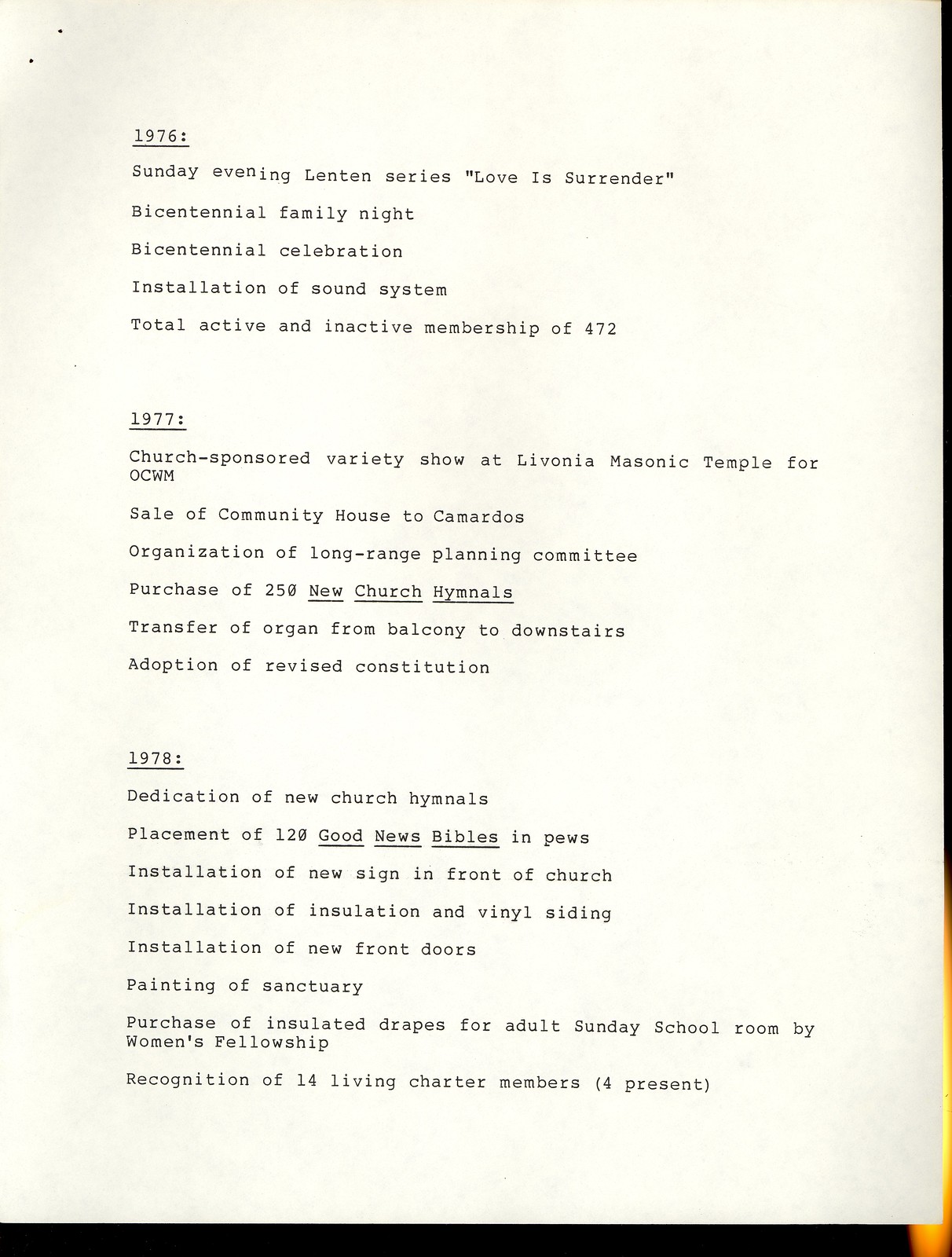The image is of an aged, off-white piece of paper, resembling a historical planner page for a religious community, featuring a chronological log of significant events and activities from 1976 to 1978. The year "1976:" is underlined at the top. Below it, the events listed include the Sunday evening Lenten series titled "Love is Surrender," Bicentennial Family Night, a Bicentennial Celebration, installation of a sound system, and a recorded total active and inactive membership of 472.

The section for "1977" includes a Church Sponsored Variety Show at the Livonia Masonic Temple for OCWM, the sale of the Community House to an organization called Comrados, the organization of a Long-Range Planning Committee, the purchase of 250 new church hymnals, the transfer of an organ from the balcony to downstairs, and the adoption of a revised constitution.

For "1978," the documented events are the dedication of the new church hymnals, placement of 120 Good News Bibles in pews, installation of a new sign in front of the church, installation of insulation and vinyl siding, installation of new front doors, painting of the sanctuary, and the purchase of insulated drapes for the Adult Sunday School Room by the Women's Fellowship. Additionally, there was recognition of 14 living charter members.

The paper also features a noticeable black strip along the bottom and a smaller strip on the right side, with a gold light shining through around the bottom right corner of the image, hinting at the document's age and the reverential care with which it has been preserved.